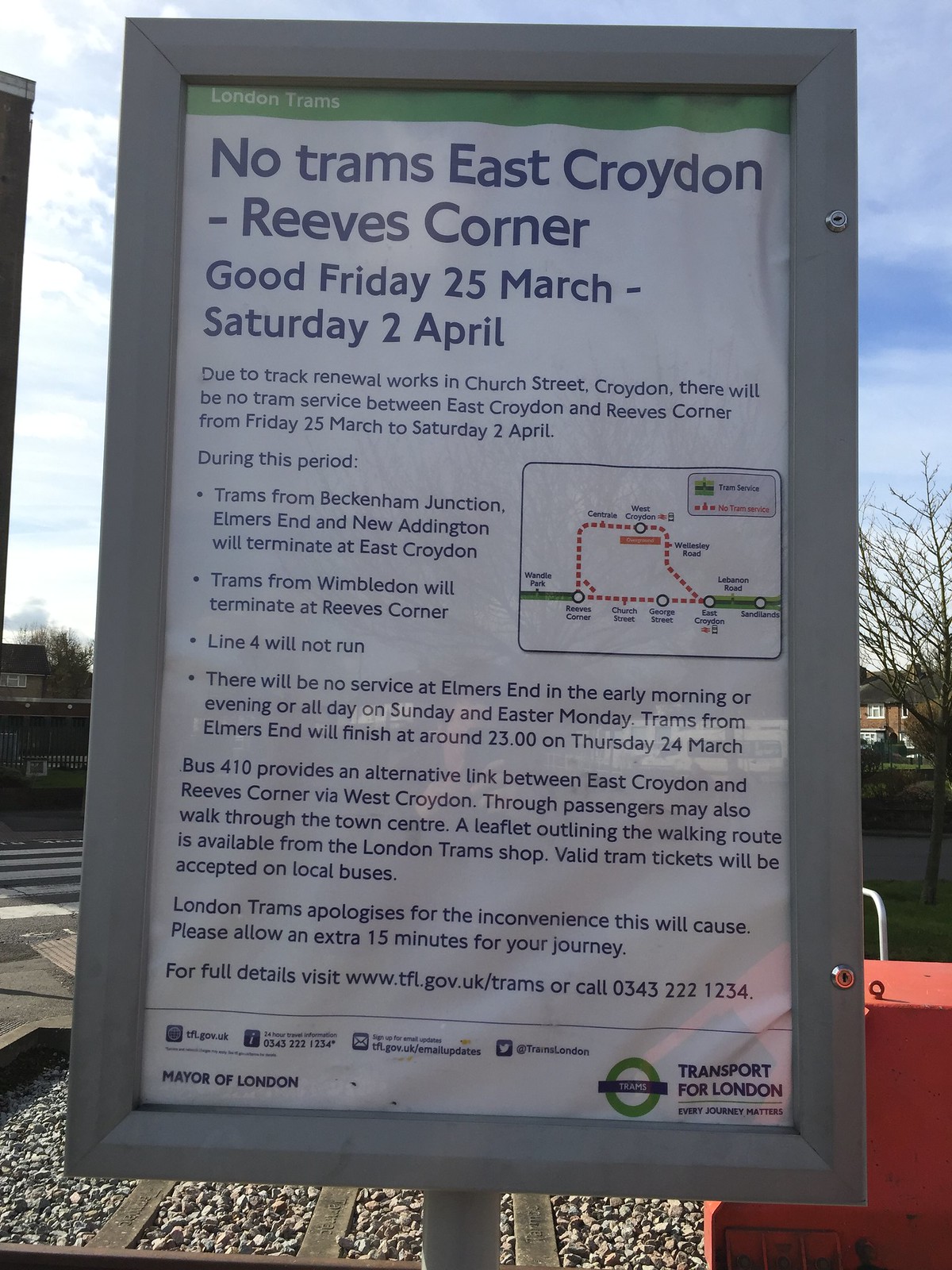The image depicts an informational notice board encased in a metal frame with a glass panel, secured by two locks—one on the top right corner and another towards the bottom left. The board features a large white poster with multiple lines of blue text, informing the public of tram service disruptions. The text reads:

"No trams East Croydon to Reeves Corner. Good Friday, 25 March to Saturday, 2 April. Due to track renewal works in Church Street, Croydon, there will be no tram service between East Croydon and Reeves Corner from Friday, 25 March to Saturday, 2 April. During this period, trams from Beckenham Junction, Elmers End, and New Addington will terminate at East Croydon. Trams from Wimbledon will terminate at Reeves Corner. Line 4 will not run. There will be no service at Elmers End in the early morning or evening. Additionally, trams from Elmers End will end at 2300 hours on Thursday, 24 March. Bus 410 provides an alternative link between East Croydon and Reeves Corner via West Croydon. Through passengers may also walk through the town center, with walking route leaflets available from the London Tram Shop. Valid tram tickets will be accepted on local buses. London Trams apologizes for the inconvenience this will cause. Please allow an extra 15 minutes for your journey. For full details, visit www.tfl.gov.uk/trams or call 0343-277-1234."

The poster is bordered by a grey wooden frame and is mounted on a grey post, possibly located at a train station or tram stop. At the top of the poster, a green banner is present, indicating "London Trams." The lower left corner features the "Mayor of London" label, while the lower right corner displays the Transport for London logo, a green circle with a blue stripe. The background appears to be gravel, suggesting the notice board is situated outside.